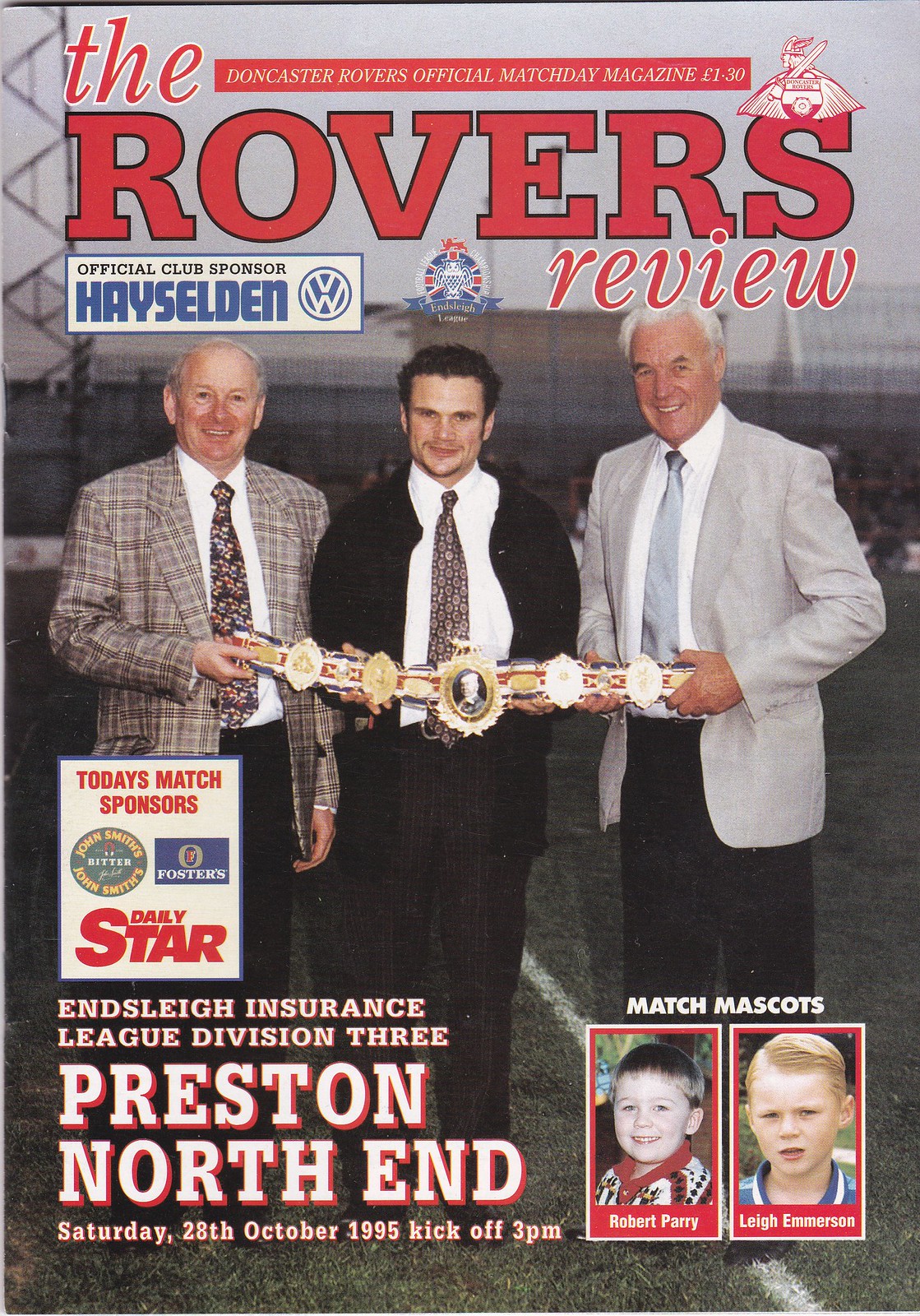The magazine cover titled "The Dover Rovers Official Match Day Magazine, L1-30 Rovers Review" features a central photograph of three men standing inside a dimly lit stadium. The trio consists of a young man in the center flanked by two older men. All are dressed in suits, each holding a decorative belt adorned with medals near their waists. The man on the left, slightly balding with gray hair, wears a checkered brown suit jacket, black pants, and a tie. The younger man in the middle sports a black suit jacket, black pants, and a brown tie, while the older man on the right has a gray jacket, blue tie, and black pants. The cover also includes various sponsor details: "Official Club Sponsor, Hayes Selden" and "Today's Match Sponsors, Daily Star." Additional sponsor icons mentioned are Foster's Beer and John Smith. The bottom of the cover notes the event details: "Inslee Insurance League, Division 3, Preston North End, Saturday, 28th October 1995, kickoff, 3pm." In the lower right corner, images of two little boys labeled as "Match Mascots" are displayed, naming them Robert Perry and Lee Emerson.